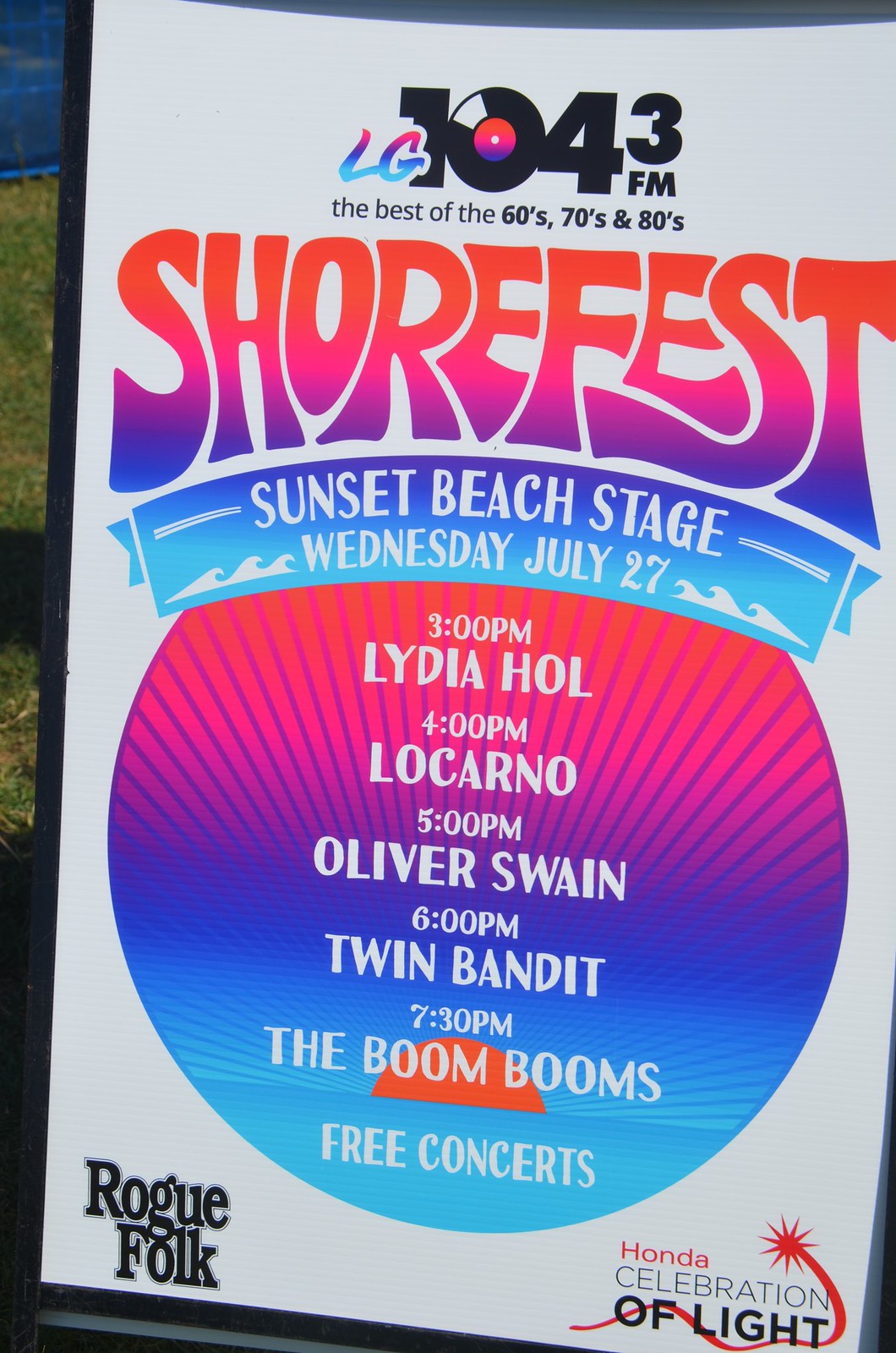This tall rectangular sign, bordered with black plastic, occupies most of the image, leaving only a glimpse of green grass and a blue fence in the top left corner. The sign’s background is entirely white. At the top, a logo in bold black letters reads "104.3 FM," with the 'O' creatively designed as a vinyl record. Above this logo, "LG" is displayed in neon-colored pink, purple, and blue letters. Beneath the frequency, the slogan "The best of the 60s, 70s, and 80s" is prominently placed. Below the slogan, "Shorefest" emerges in a large, vibrant gradient font shifting from orange to purple, embodying a hippie aesthetic with its playful lettering.

Further down, a section detailing event information is bordered by a blue banner, listing performers scheduled for the Sunset Beach Stage on Wednesday, July 27th. The performance lineup, in a sunburst pink and blue circle, includes: Lydia HOL at 1 PM, Locarno at 4 PM, Oliver Swain at 5 PM, Twin Bandit at 6 PM, and The Boom Booms at 7 PM. A note at the bottom of this section highlights that these are "Free Concerts."

In the bottom left corner, the words "Rogue Folk" appear. On the lower right, "Honda Celebration of Light" is printed, accented by a sunbeam and a red line crossing through the text.